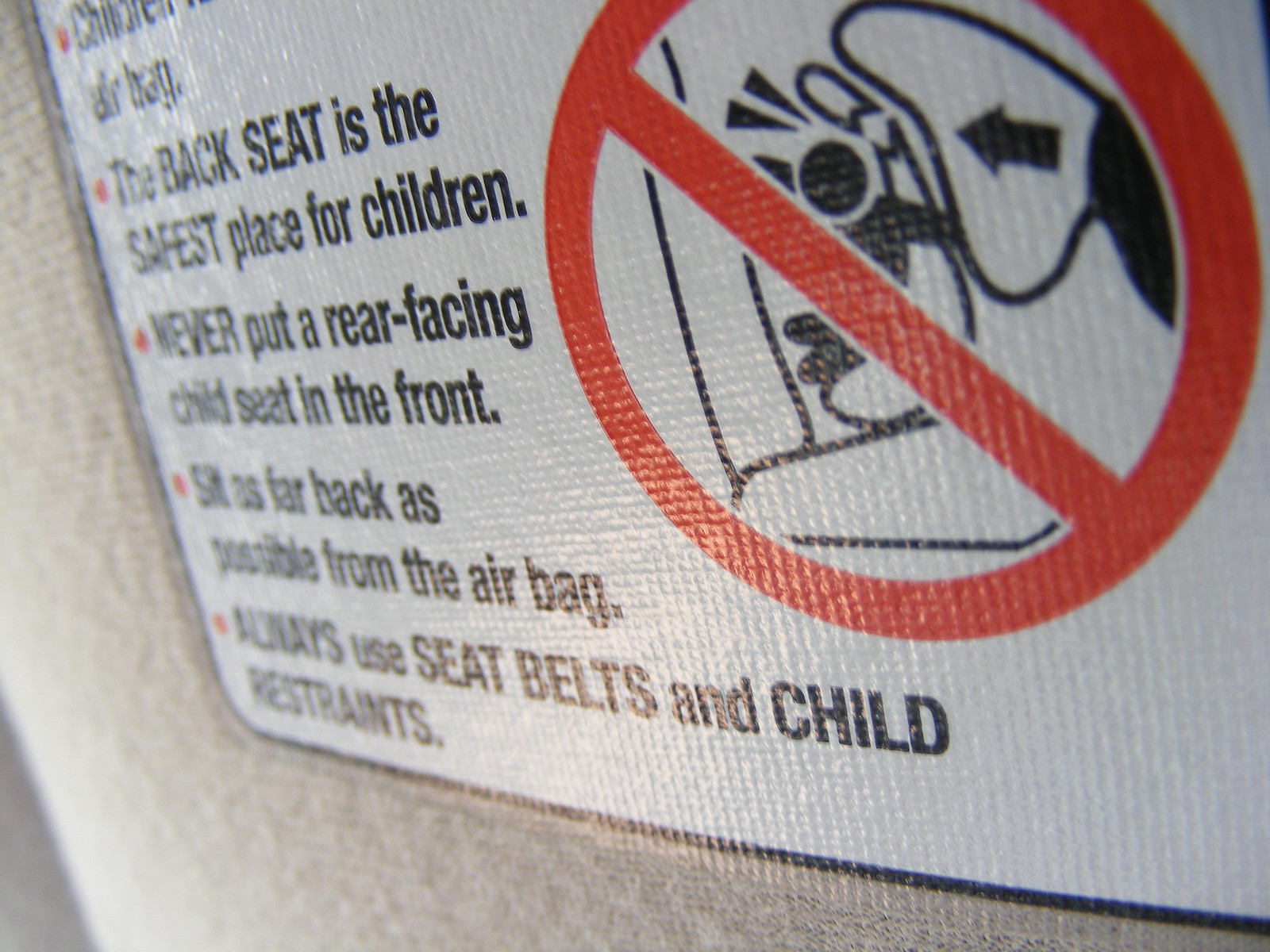This is a close-up photograph of a warning sticker affixed to a car visor. The sticker appears to be white and plasticky, placed on a textured, cream-colored surface, possibly a vehicle's interior. It prominently features a red circle with a diagonal line through it, depicting a child in a car seat positioned in front of an airbag, indicating this setup is unsafe. The left side of the sticker contains several red bullet points with safety instructions in black text, advising: 

1. The back seat is the safest place for children.
2. Never put a rear-facing child seat in the front.
3. Sit as far back as possible from the airbag.
4. Always use seat belts and child restraints.

The image is angled, causing some parts of the text to be difficult to read, but these key safety messages are clear.